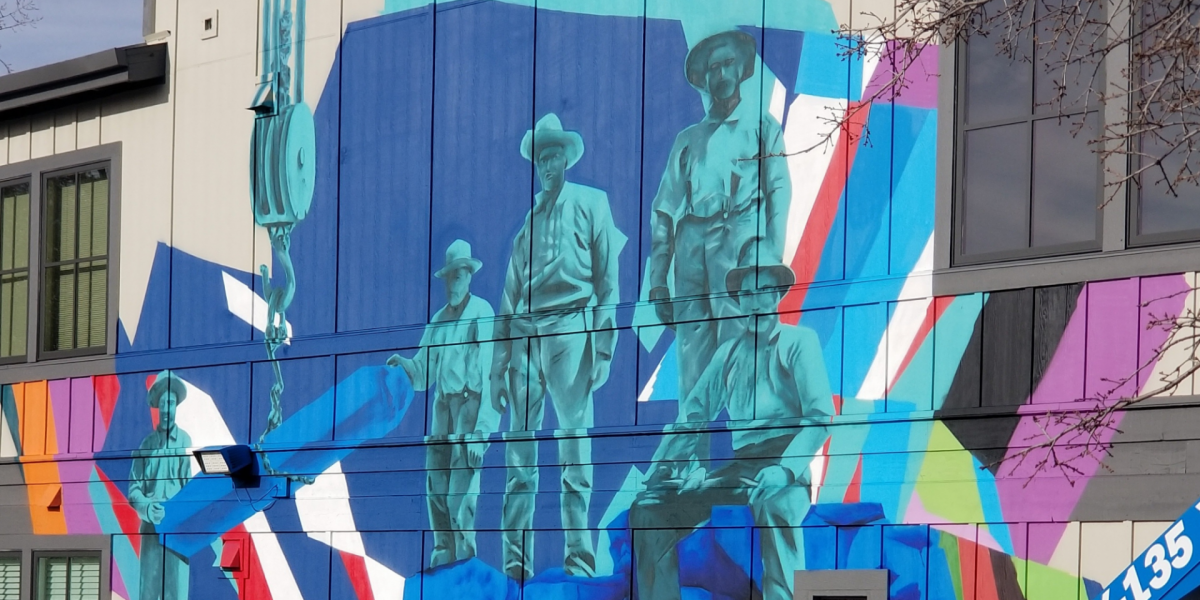The image showcases an outdoor mural painted on the side of a predominantly white building, with a colorful background featuring shades of blue, turquoise, and various streaks of orange, lavender, red, yellow, green, and brown. Centrally positioned on the building, the mural illustrates five men, depicted in teal/turquoise. These men appear to be middle-aged or older, dressed in old-style construction attire, including hats, long-sleeved shirts, overalls, and jeans. The workers are engaged in construction activities: one man is off to the side on the left, holding a blue cylindrical object along with another man from the central group, suggesting a collaboration possibly aided by a crane. The mural is framed by office windows on both sides; the windows on the right are dark and unblinded, while those on the left feature dull yellow blinds.